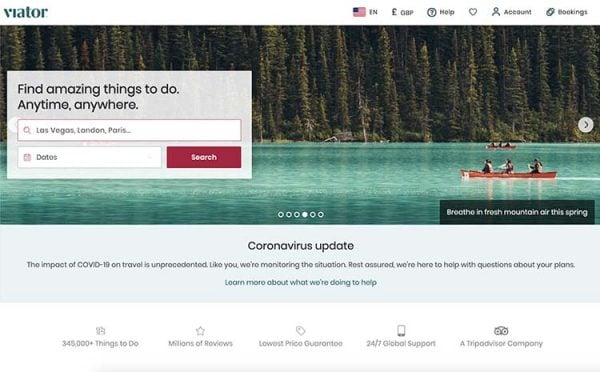In the upper left corner, the text "BIATOR" is prominently displayed. On the upper right side, various icons are visible: an American flag, "EN" for English, currency symbols for pounds (GBP), a question mark inside a circle for help, a heart, and a ribbon, followed by the text "Account" and "Booking."

Below these elements is a serene photograph depicting a turquoise lake or river, over which two orange kayaks glide peacefully. The kayaks are manned by people enjoying the water. In the background, a dense forest of dark green pine trees stretches across the landscape. 

On the left side of the image, a rectangular banner spans horizontally, shaded in grey and black. It invites viewers with the phrase, "Find amazing things to do anytime, anywhere." Beneath this are two search fields: one suggesting locations such as "Las Vegas, Paris, London," and another dedicated to dates. A bold red button marked "Search" in white text completes the banner.

At the bottom right of the photograph, the caption "Breathe in fresh mountain air this spring" encourages seasonal adventure. Below this, a middle-aligned notice reads, "Coronavirus Update: The impact of COVID-19 on travel is unprecedented. Like you, we are monitoring the situation."